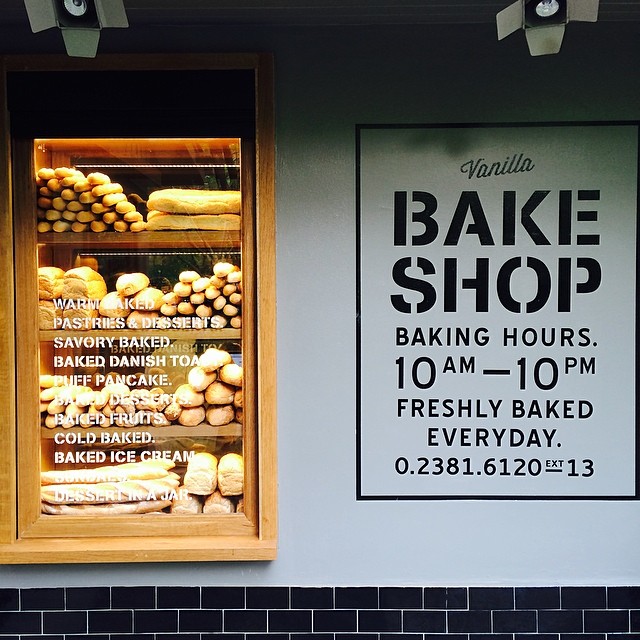This image depicts the inviting facade of the Vanilla Bake Shop. On the left, there is a well-lit display window, encased in wood and glass, showcasing an array of fresh baked goods meticulously organized on four shelves. The assortment includes various types of bread such as normal loaves, long loaves, small baguettes, and rye loaves. The shelves are adorned with white font labels listing items like Warm Baked Pastries and Desserts, Savory Baked, Baked Danish, Toast, Puff Pancake, Baked Fruits, Cold Baked, Baked Ice Cream, and Dessert in a Jar.

On the right side of the image, a prominent vertical rectangular sign with a black outline catches the eye. The sign reads "Vanilla" in a cursive navy blue font at the top, followed by "Bake Shop" in bold, uppercase letters. Below this, the sign details the baking hours, 10 a.m. to 10 p.m., and proudly announces "Freshly Baked Every Day." At the bottom, a contact number, 0.2381.6120EXT13, is displayed. The background of the facade features a light blue wall, complemented by a pattern of navy-colored bricks at the bottom, enhancing the overall charm and appeal of the shop.